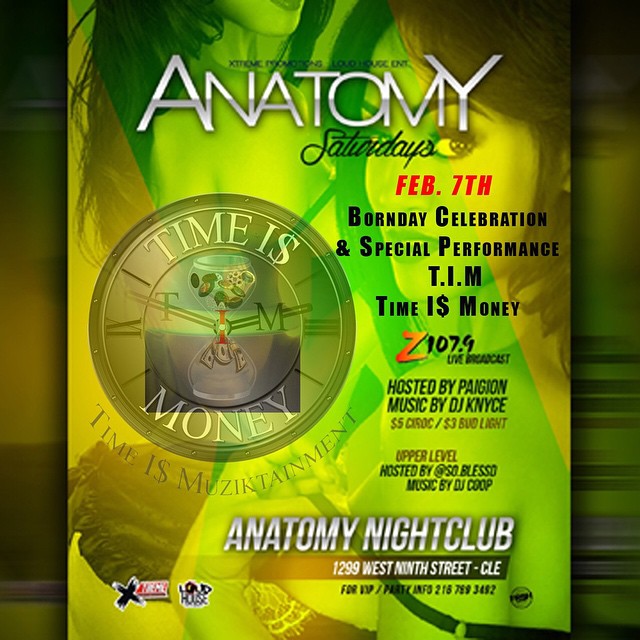The image is an advertisement poster for an event at Anatomy Nightclub, located at 11299 West 9th Street, Cleveland. The poster features a green, gold, and red background and prominently displays images of two scantily clad women. At the top, "Anatomy" is written in white and light gray text, followed by "Saturdays" in black cursive. The event is set for February 7th, with the text "Born Day Celebration and Special Performance: T.I.M. - Time is Money" in red and black. The poster also highlights a Z107.9 live broadcast hosted by Pagion, with music by DJ Nice, and mentions $5 Ciroc and $3 Bud Light specials. The upper level of the nightclub will be hosted by AxoBlessed with music by DJ Coop. Additional details include the club's call-to-action for VIP and party information at 216-789-3492. A notable round logo features an hourglass with coins and dollar bills, encapsulated by the phrase "Time is Money," alongside the words "Time is Music Tainment." Two small logos are positioned in the bottom left corner, and a larger logo appears in the middle left section of the poster. This event is presented by Extreme Promotions and Loud House ENT.